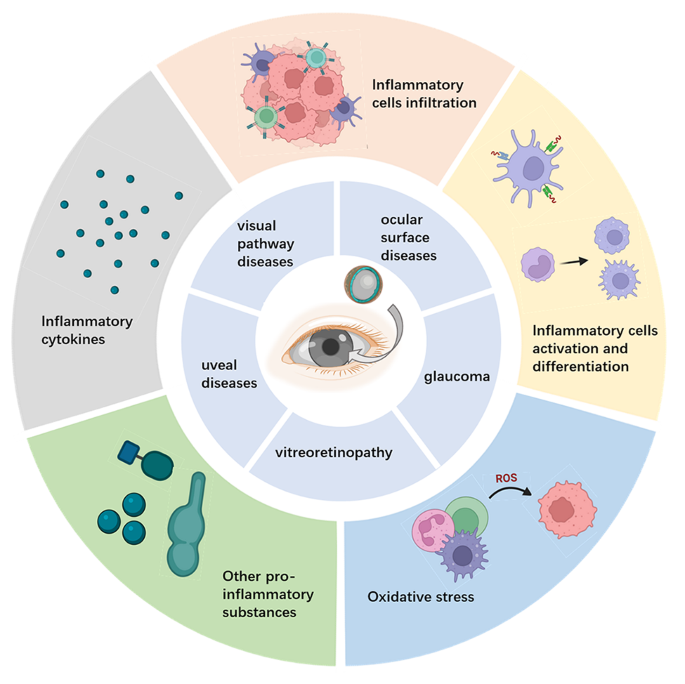The image is a detailed circular chart focusing on various eye diseases and related factors. At the center of the chart is an illustration of an eye, featuring a white circle with a black pupil and a gray iris. Above the eye, a gray circle connects with an arrow pointing downward to the eye. Surrounding the central eye illustration is a light blue or grayish ring divided into five sections, each labeled with black writing such as "visual pathway diseases," "glaucoma," "ocular surface diseases," "vitreoretinopathy," and "uveal diseases."

Encircling this ring is a thin white band, followed by an outermost layer divided into five colored segments, each highlighting different pathological factors associated with eye diseases. These segments, colored in pink, light orange, light blue, light green, and lavender, contain images and labels like "oxidative stress," "other pro-inflammatory substances," "inflammatory cytokines," "inflammatory cell infiltration," and "inflammatory cell activation and differentiation." The diagram serves as a comprehensive visual representation of the various diseases and pathological processes affecting the human eye.